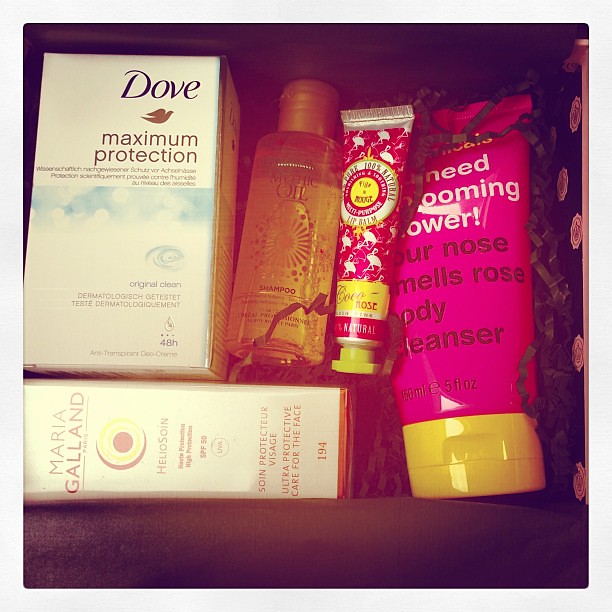The image depicts an assortment of health and beauty products meticulously arranged, possibly within a dresser drawer or a box. The background is predominantly dark with some light glimmers adding contrast. Central among the items is a white box displaying "Dove" in black font and a gold dove symbol. It prominently features the words "Maximum Protection" also in gold, followed by difficult-to-read but important texts like "Original Clean" and "Dermatologist Tested" suggesting 48-hour protection in blue font.

To the right of the Dove box stands a shampoo bottle with a gold lid containing a golden liquid identified as "Mythic Oil." 

Adjacent to the shampoo are two pink squeeze bottles. The first has distinctive white flamingo graphics and a yellow lid, adorned with various colored circles including yellow, white, and pink. This bottle possibly denotes a nature-based product, emphasizing natural ingredients.

The second pink squeeze bottle is noted for text like "Our Nose Smells Rose Body Cleanser," which suggests a floral scent, and appears to be sized similarly to the shampoo bottle.

Finally, a tilted white box labeled "Maria Galland" in black font rests on the far left. This box includes detailed brown text possibly naming Heliosophia and promoting ultra-protective facial care marked as "Soin Protector Visage 194."

Each product is offset by the dark padding and black base of the container, enhancing the visibility of their labels and designs.